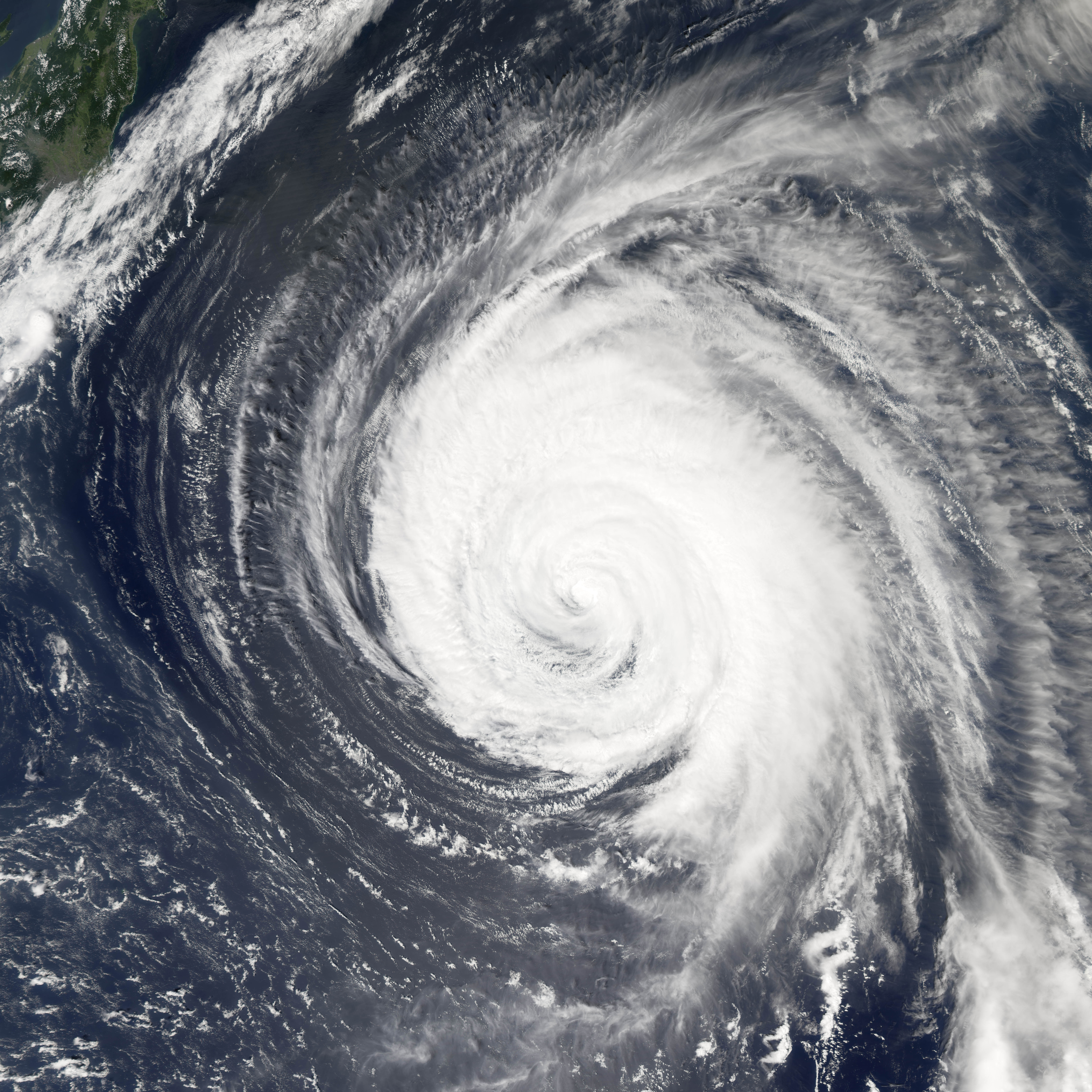The image is a detailed color satellite photograph capturing an impressive and massive hurricane over a blue ocean. The focal point of the image is a dense, white, swirling mass of clouds centered around the hurricane's well-defined eye. This central swirl is very tight and bright, indicating the storm's powerful core, while the outer arms of the hurricane are fainter, less dense, and more dispersed. The clouds exhibit a counterclockwise rotational pattern, typical of such storms in the Northern Hemisphere. In the top left corner of the image, there is a patch of green land, which contrasts sharply with the surrounding vast expanse of swirling ocean. The photograph emphasizes the dramatic and spiraling movements of the storm, characterized by the churning, frothy water and textured waves. The satellite view provides a realistic and detailed perspective, making the image both informative and visually striking.